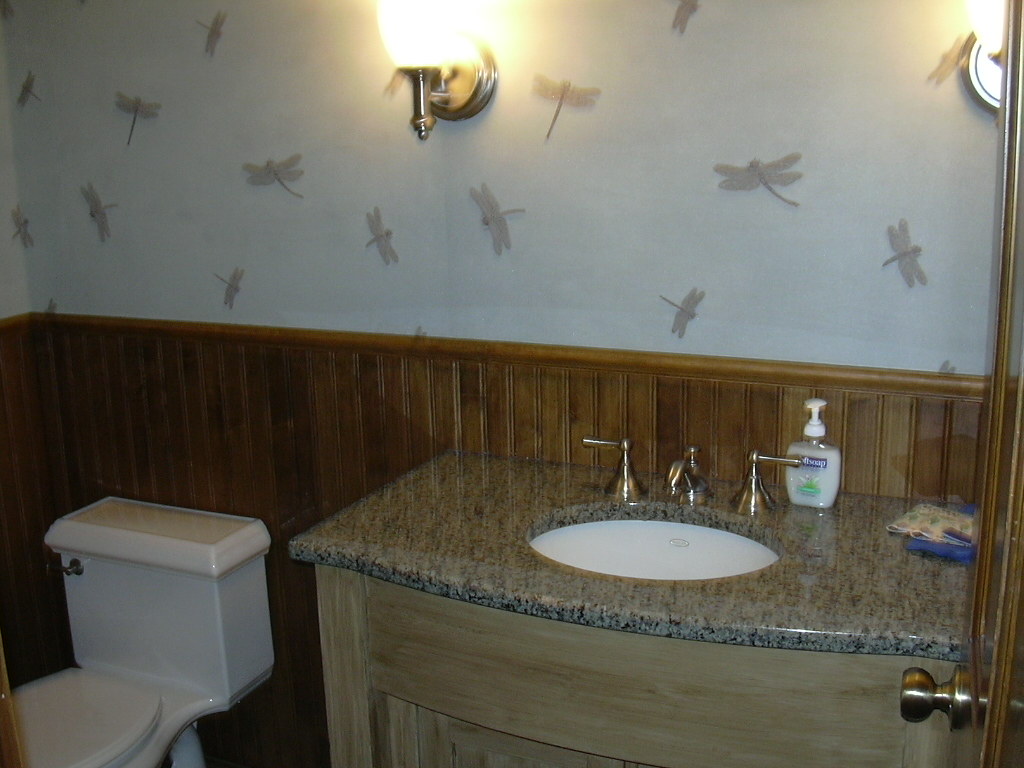This photograph offers a comprehensive view of a modestly-sized, elegantly designed bathroom, captured from the entrance. The room is wider than it is tall, creating a sense of spaciousness. On the right, the door is partially open, inviting the viewer into the space. The back wall is strikingly divided horizontally. The top half is painted white and adorned with subtle, randomly patterned light gray dragonfly illustrations, lending an air of tranquility. Two wall sconces, turned on, illuminate the room; one is positioned slightly left of center, while the other is in the far upper right corner, almost out of frame. 

The lower half of the back wall features vertical wooden slats, contributing a touch of rustic warmth to the room. 

To the left of the photograph, a modestly sized toilet with a closed lid sits unobtrusively. On the bottom right, a large vanity takes center stage. It includes a granite countertop, which hosts a modern faucet with two knobs and a soft soap dispenser. The vanity features a circular basin with a white bowl, exuding a clean, minimalist aesthetic. Notably, the bathroom lacks a mirror and towel racks, allowing the space to remain uncluttered. The only visible fixtures are the toilet, the vanity, and the wall sconces, which together create a serene and functional environment.